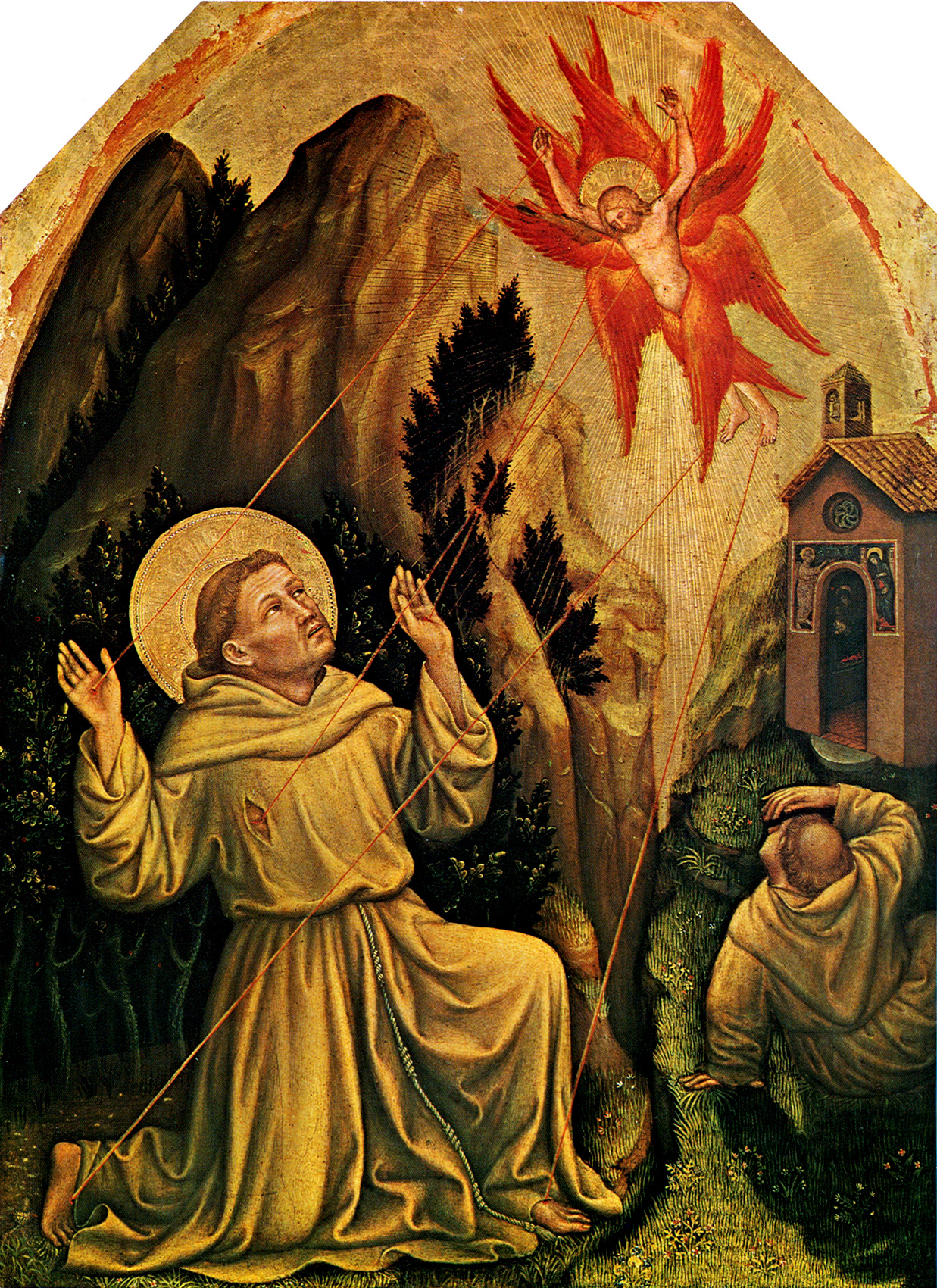This tall, rectangular painting is a richly textured religious artwork, possibly a textile or weaving, notable for its intricate details and vibrant colors reminiscent of traditional stained glass. The central scene is dramatic and awe-inspiring, featuring two friars and a celestial vision.

In the painting's foreground, a friar in a greenish-brown, baggy robe kneels on one knee with his hands raised in reverence. His gaze is fixed upward towards the top right corner, where an ethereal, crucified figure of Jesus hangs in a sky filled with a multitude of fiery red and orange wings. This Jesus figure, seemingly enveloped in these bright wings, adopts a crucifixion pose, with crucifixion wounds evident on his body. From these wounds, thin, red, laser-like beams pierce down to the kneeling friar below, striking at his hands, feet, and side, mirroring the stigmata. Both the friar and Jesus have gold medallions, or halos, behind their heads, symbolizing their holy nature.

To the side, another friar, distinguished by his shaved patch typical of a friar's tonsure, lays on the grass with his back facing the viewer. He shields his eyes from the divine brightness, looking up at the miraculous vision amidst the overwhelming radiance.

In the backdrop, an open door reveals a small, rustic sanctuary or church with a clay tile roof, a compact bell tower, and a small stained-glass window. To the left of the kneeling friar is a looming mountain, adding to the dramatic scenery of this celestial event. The painting captures a moment of profound spirituality, illustrating a divine intervention or miraculous occurrence that leaves its earthly witnesses in a state of awe and disbelief.